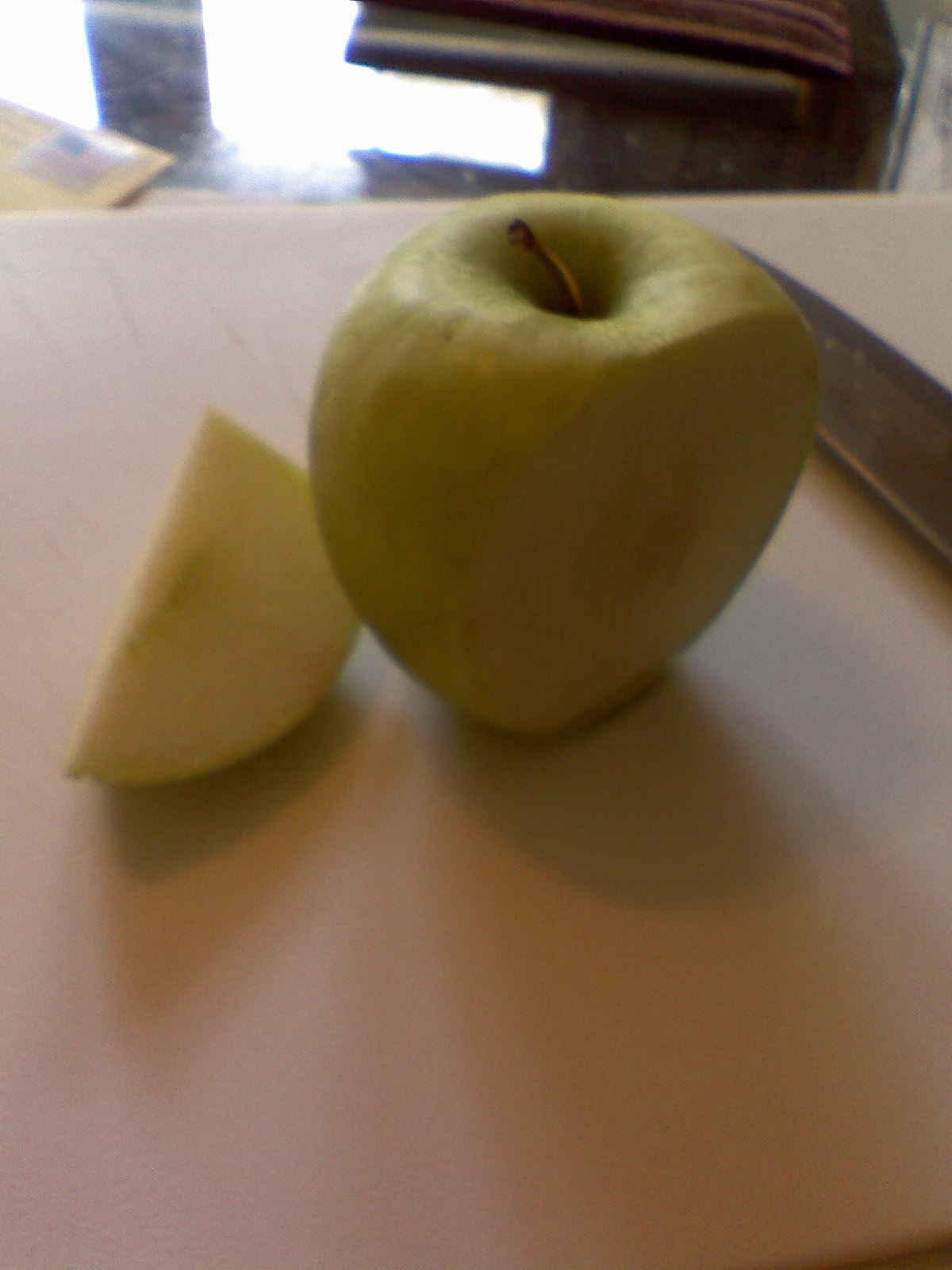The photograph is a rectangular image with the left and right sides being longer than the top and bottom sides. It prominently features a green apple positioned at the center, with approximately one-fourth of the apple having been sliced away, revealing the white flesh and brown core. Portions of the exposed white flesh have started browning. The cut side of the apple points towards the left of the photo, and the apple is placed on a white plastic cutting board that shows several notches and cuts.

To the left of the apple lies an apple wedge, clearly a segment from the sliced section. This wedge displays a thin green strip of the core at its center, white flesh, and green skin, along with a small brown spot on its edge. In the top right corner of the photograph, a silver curved cutting knife's blade is visible, adding context to the slicing process.

The cutting board itself is situated on a highly reflective surface, resembling glass. Adding an unexpected element to the composition, there is a yellow envelope with an American flag stamp in the top left corner of the image.